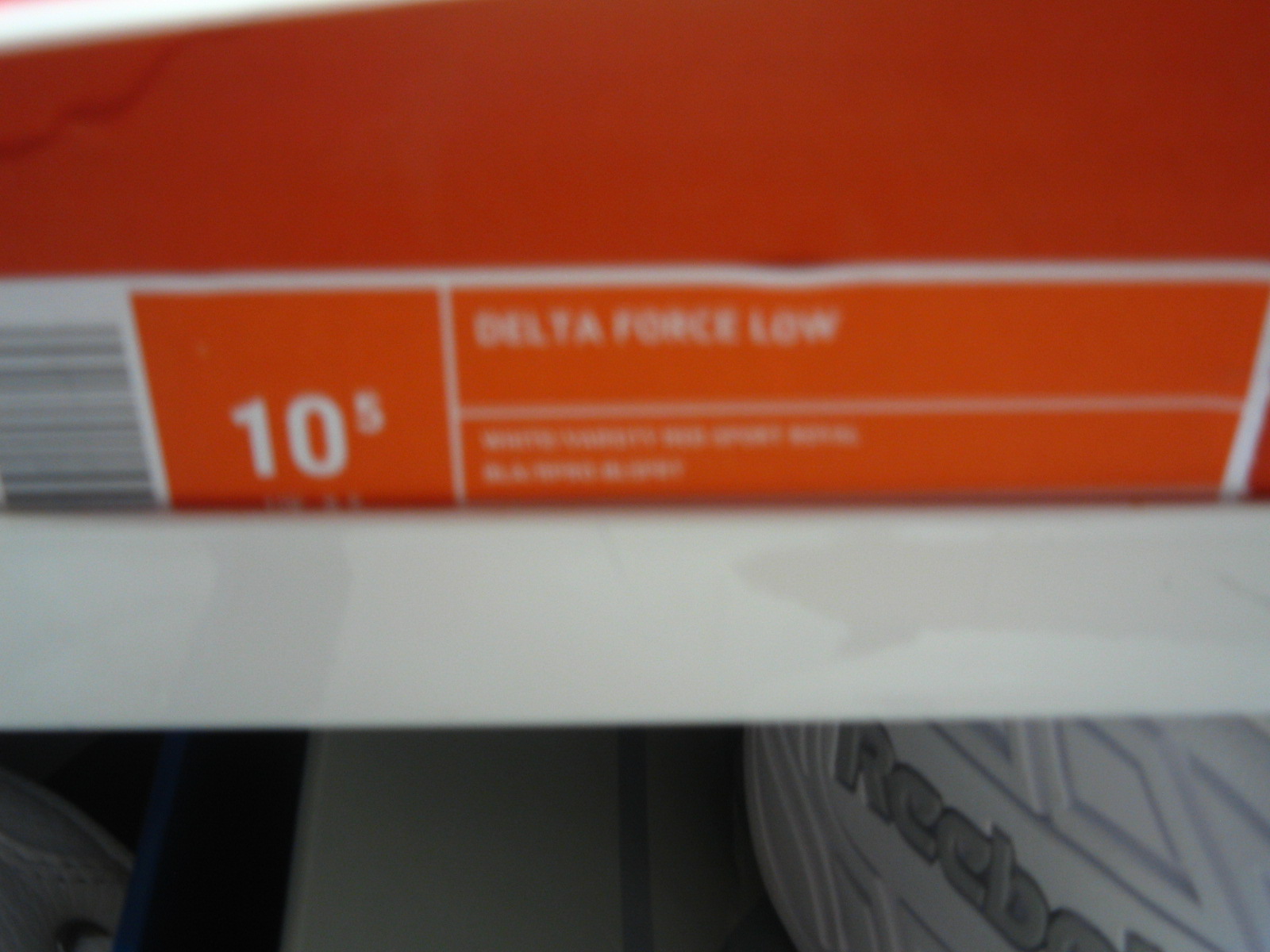The image is an indoor photograph focusing on a shoe box, which appears blurry and out of focus. The box itself is predominantly orange with white accents. Despite the blurriness, the words "Delta Force Low" can be discerned in white lettering on the box. Below this, there is additional writing that is too out of focus to be legible. The box also features the numbers "10" and "5" in white, each enclosed within separate white-bordered boxes. A barcode is present as well. Below the main orange section of the box is a white stripe. Beneath this stripe lies part of a shoe sole, which is white and partially reveals a logo reading "Reebok" in silver letters.